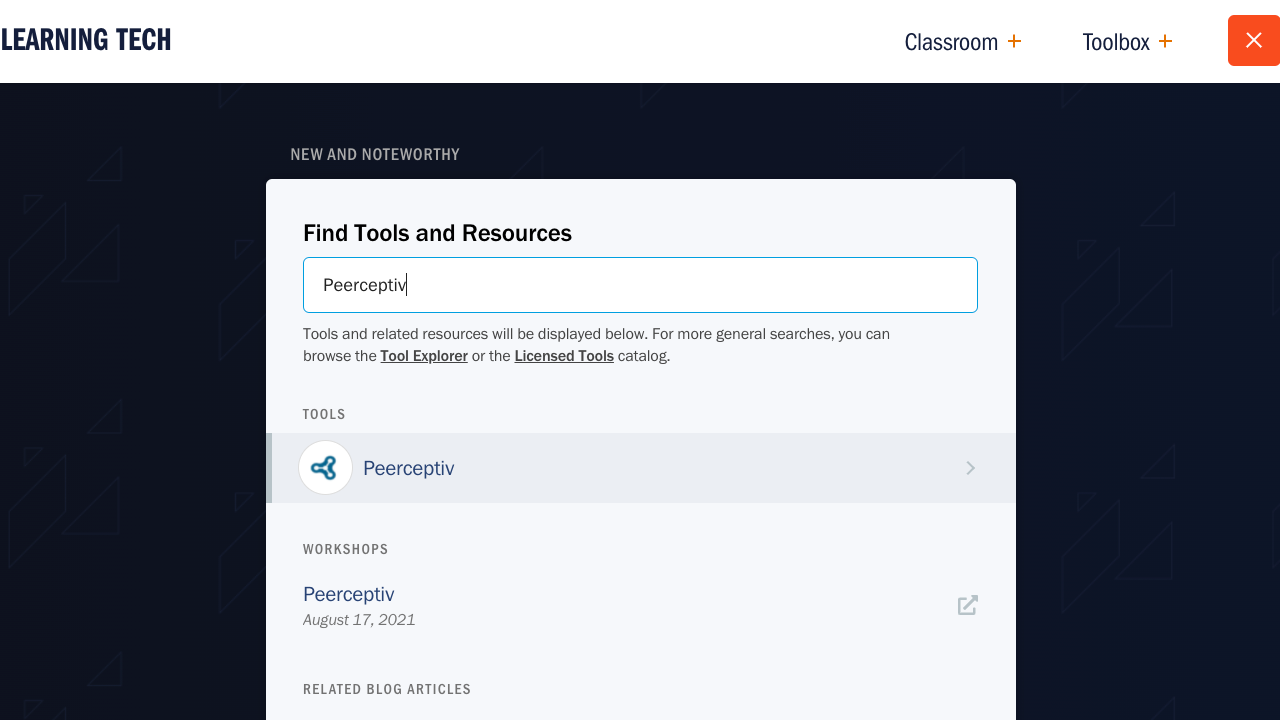The descriptive caption for the given image can be formulated as follows:

---

The image showcases a webpage titled "Learning Tech" in bold, black, uppercase letters at the top. Directly beneath this header, there is a clickable button labeled "Classroom," accompanied by an icon, possibly for adding new content or navigating to a different section. To the right, there's a red button with an X, presumably for closing the interface.

In the center of the page, a user appears to be in the process of typing "PEERCEPTIVE" into a search bar designated for finding tools and resources. The incomplete text in the search bar reads "P E P E E R C E P T I V," with the cursor indicating an ongoing input.

Displayed below the search bar is a message indicating that tools and related resources will appear based on the search input. It also mentions that users can browse through a "Tool Explorer" or view a "Licensed Tools" category for more general searches.

Further down, the page features a section about a "Peerceptive Workshop" that was scheduled for August 17th, 2021. This section includes a related blog article link, likely providing additional information about the workshop. Additionally, it offers options to sign up for training sessions or forward the workshop details to others.

Overall, the image gives a detailed look at a user interface designed to assist users in finding educational tools and registering for relevant training workshops.

---

This caption offers a comprehensive description of the image, covering all key elements and their functions.